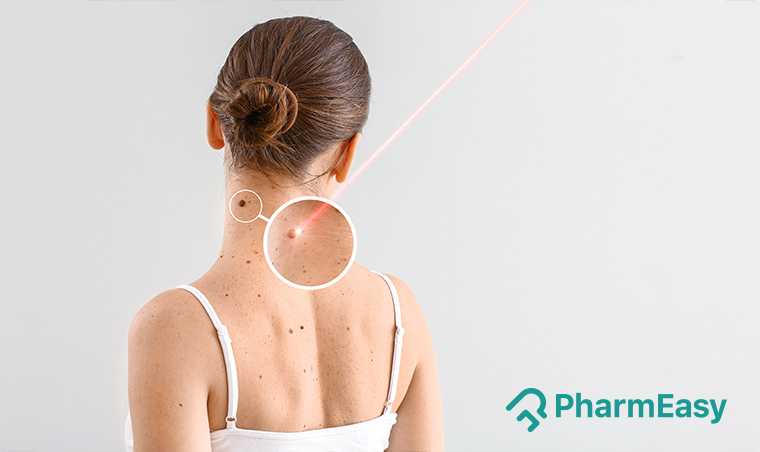In this advertisement image, we see the back view of a woman with dark brown hair tied up in a bun. She is wearing a white tank top with string shoulder straps, which exposes part of her back and neck. The background is light grey. Highlighted in the image is a close-up of a mole on the back of her neck, surrounded by an edited circle. A red laser light is depicted as targeting this mole from the top of the image. Another smaller circle magnifies another mole nearby. At the bottom right corner, the words "Farm Easy" are written in green, accompanied by a logo, suggesting it's a pharmaceutical advertisement aimed at mole removal.